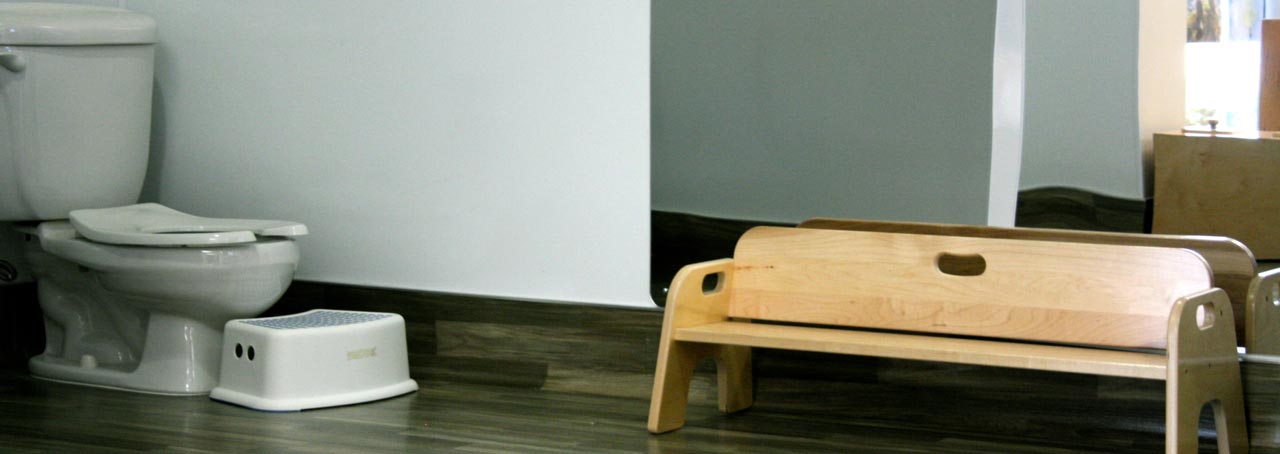This bathroom scene is captured in a panoramic-style photograph. On the left side, a white porcelain toilet stands prominent, with a small, curved white plastic step stool featuring a textured gray lid positioned in front of it, likely used by toddlers for assistance. The toilet sits on a dark, wooden paneled floor that extends slightly up the wall before transitioning to a clean, white surface. On the right side of the image, a short, wide wooden bench, about the same height as the toilet, is placed in front of a wall-mounted mirror, reflecting the bench and a wooden table in the background. The wooden bench is equipped with handles, suggesting it might be a step stool for children. The combination of the dark floor, white walls, and wooden furnishings creates a harmonious and functional children's bathroom area.